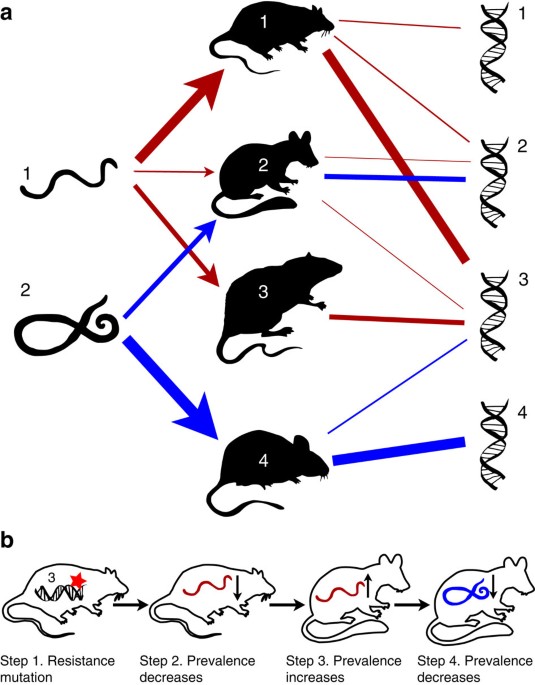The image depicts an educational chart with a predominantly white background, illustrating steps in a biological process related to mice and resistance mutation prevalence. At the top of the chart, there are two sections labeled A and B. Section A includes three rows and three columns. The first column contains silhouettes numbered 1 and 2, resembling worm-like or snake-like structures. The second column shows silhouettes of mice, each labeled 1 through 4. The third column features silhouettes labeled A and B, also numbered 1 through 4. Red and blue arrows, along with lines of the same colors, connect these silhouettes.

In section B, located at the bottom of the chart, four mice silhouettes are arranged in a row from left to right. Each mouse is numbered and associated with specific text indicating steps: Step 1 is labeled "resistant mutation," Step 2 "prevalence decreases," Step 3 "prevalence increases," and Step 4 "prevalence decreases" again. Arrows between these silhouettes point towards the right, suggesting a sequential process. 

The mice silhouettes contain colored lines and shapes, including white, red, and blue squiggly lines, and a notable red star in one of the mice in the bottom left. Overall, the objects in the image are well-organized but not strictly centered. The chart utilizes a combination of black, white, red, and blue colors and features text written in black. This digitally created chart effectively depicts the steps involved in the mutation and prevalence of resistance in mice.